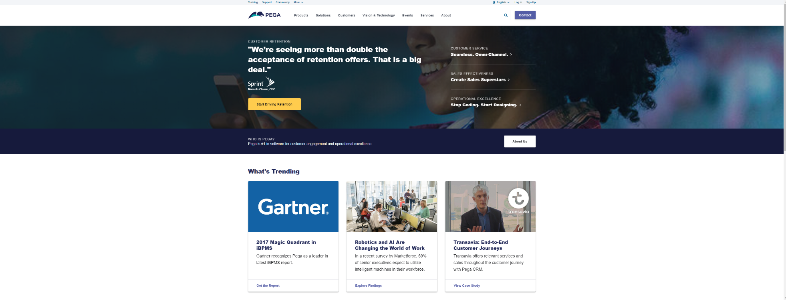The screenshot captures a computer screen with a predominantly white background. At the top center, there's a stylish teal and purple logo accompanied by a name. Below the logo, several categories or clickable tabs are organized in a horizontal layout.

Beneath these tabs is a wide but shallow banner image. This image features a gradient background transitioning from teal to pastel, jewel-like hues, with a soft, blurred effect. Within the banner, a woman with curly black hair and a collared shirt is prominently smiling and glancing to the left, seemingly looking at a phone. Her cheerful expression highlights her nose and teeth.

Superimposed on this banner image, there's a white text overlay, although the specific words are unreadable. Additionally, on the left side (yet still within the central area of the page), there's a small yellow button inviting user interaction.

Further down the page, three evenly spaced boxes present a "What's Trending" section. Each box includes an image at the top with accompanying descriptive text beneath. The first box showcases a blue square with the word "Gardner" inscribed. The middle box features an image of numerous people inside a skyscraper, while the box on the right displays a man in the midst of speaking or addressing an audience.